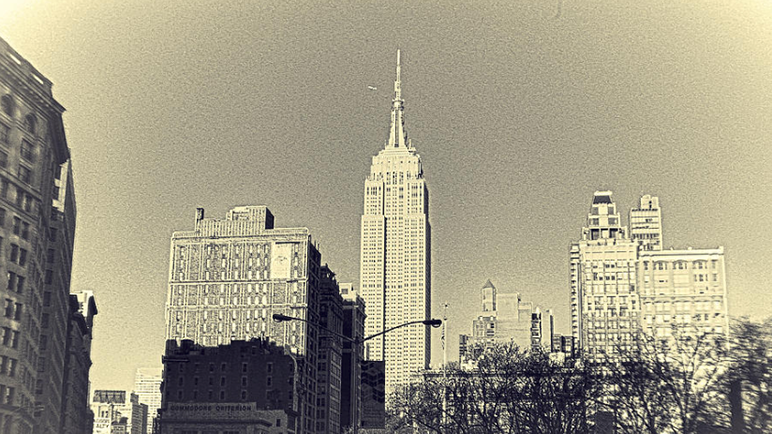This black and white photograph, likely of New York City, is taken from street level and showcases an intricate urban composition dominated by a towering skyscraper in the center, which closely resembles the Empire State Building. It stands approximately 40 stories tall with eight windows across each floor and culminates in a pointed needle at the top. On the left side, a large building covered in windows extends vertically down the edge of the photo. In the far background, there is a smaller white building to the right, followed by a flat-fronted building with rows of windows, flanked by two more buildings behind it. 

To the right of the central skyscraper, another smaller building stands further in the background. Closer to the foreground on the right, a white rectangular building with windows features an additional layer of 4 or 5 stories on top. The lower portion of the image reveals a line of trees with sparse leaves and a light pole with two lights extending from its top. The lighting suggests it's morning, as the right side buildings receive direct sunlight casting significant shadows on adjacent structures, while parts of the left-side buildings remain shaded. The sky, clear and monochromatic, emphasizes the stark contrast and depth within this urban landscape.